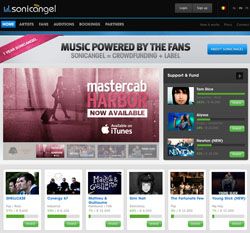Colorful square-format screenshot of the Sonic Angel website. The website's name, "sonic angel," is displayed in all lowercase white lettering with an accent mark over the letter 'A' in "angel." Six navigational tabs are located beneath the site name, with the "home" tab selected in this view.

The homepage features a prominent banner across the top that reads: "Music Powered by the Fans - Sonic Angel + Crowdsourcing + Label." This suggests the platform operates on a crowdsourcing model to gauge music's popularity and involve fans directly.

To the right and below the banner, the page showcases a series of articles about various artists and their albums. The articles include images of the artists; one image shows a performer singing into a microphone, while another highlights an artist looking directly at the camera. Additionally, there are thumbnails of album covers presumably available for purchase or streaming. 

Overall, the detailed layout of the website offers an engaging preview of content related to fan-powered music and artist promotions.